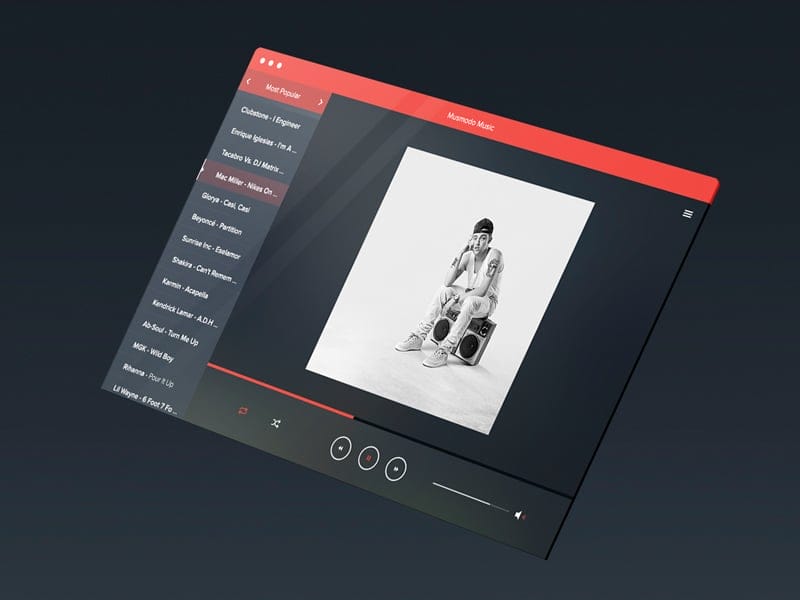**Caption:**

The image depicts a stylized web page interface set against a pure black void, giving it a 3D rendered appearance. The highlighted focal point on the page features a young white boy adorned with tattoos on both arms. He is casually dressed in jeans, a tank top, and a backward baseball cap, and is sitting atop a large 1980s-style boom box with the sound level set three-quarters high, indicating it's currently paused. The background is a pristine white, starkly contrasting the floating web page.

A prominent red bar at the top of the interface displays the name "Buzzbundo Music." On the left side, there's a list detailing some of the most popular artists, including Mac Miller, Beyoncé, Sunrise Inc, Shakira, Acapella, and Kendrick Lamar, though the text is small and somewhat challenging to read. The web page seems to function as a song selector or music organizer, branded under a name that is partially obscured but resembles "Old Modo Mando."

Overall, the design conveys a retro-modern aesthetic, merging elements of past and contemporary digital music culture.